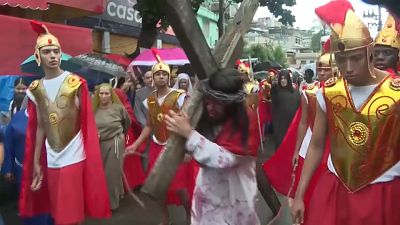The image captures a street reenactment of the Passion of the Christ, set against a bustling marketplace backdrop. Central to the scene is a character embodying Jesus Christ, clad in a blood-stained white tunic and a crown of thorns, solemnly carrying a large wooden cross. Flanking him are Roman soldiers adorned in traditional attire: gold helmets with red feathers, gold chest plates over white shirts, red robes, and golden crowns with red accents. One soldier positioned behind Jesus wields a whip. The backdrop reveals a poverty-stricken area with numerous businesses, including a visible shop labeled "Casa" on the top left and tan-gray housing on the top right. The gathering includes individuals in modern plain clothes as well as spectators lining the street, suggesting a modern-day setting. The sky is overcast, adding a somber tone to the trees and bushes dotting the scene.